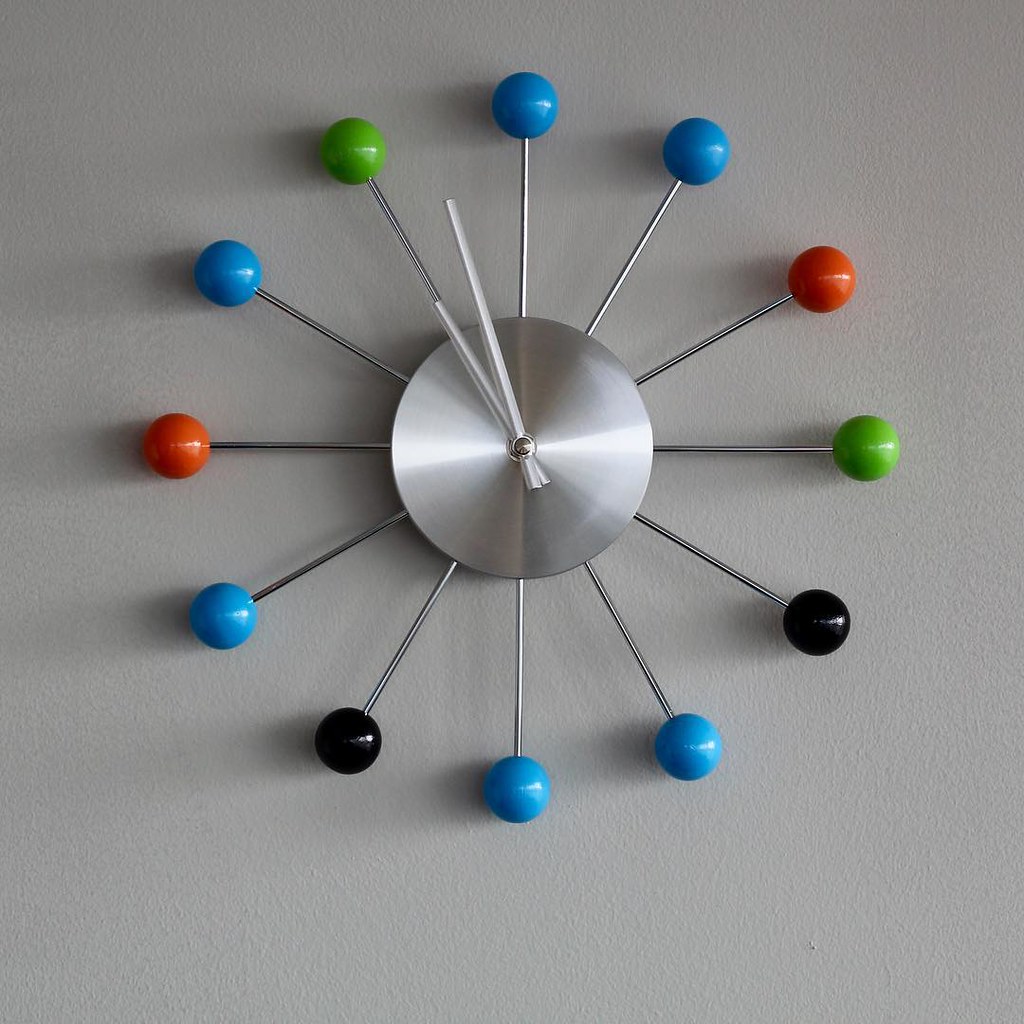This image portrays a photograph of a uniquely designed, avant-garde wall clock, set against an off-white or neutral gray background with a faint texture. The clock features a sleek, brushed stainless steel central disc devoid of numerals. From beneath this central disc, twelve slender metallic rods extend outward, each tipped with a vibrant, round colored ball. The balls, which appear in hues of blue, green, orange, and black, are positioned to signify the hour markers in a seemingly random arrangement, evoking a whimsical, retro aesthetic reminiscent of the 1960s. The clock hands, metallic in nature and possibly semi-transparent or white, extend from the disc's center, with one longer to indicate minutes and the shorter to mark the hours. This striking piece of art, resembling an abstract machine more than a traditional timepiece, captures a blend of futuristic and retro design elements.